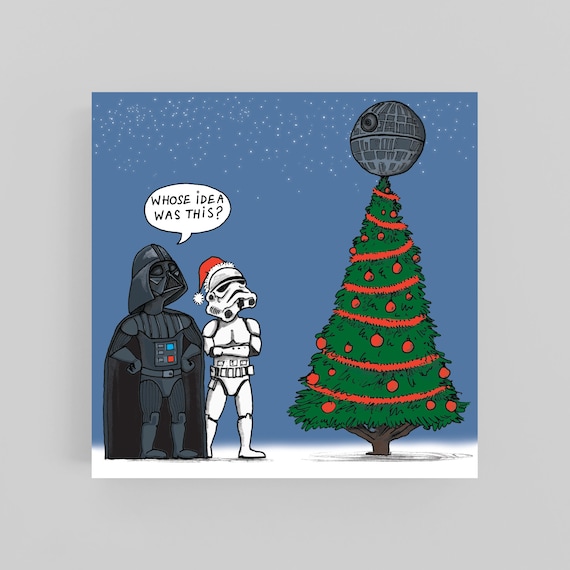This humorous cartoon comic frame features the iconic Star Wars characters Darth Vader and a Stormtrooper standing on a white floor with a navy blue background adorned with small white dots that resemble falling snow. On the left side, Darth Vader is depicted wearing his classic black outfit complete with blue and red buttons on his chest, and his signature sloping black helmet covering his face with a triangular mouthpiece. He is gazing slightly upwards and to the right. To his right stands a Stormtrooper, clad in white armor and a fully covering white helmet, topped with a whimsical Santa hat whose pom pom droops to the left. The Stormtrooper also looks upwards and to the right.

To the right of both characters is a festive Christmas tree, featuring a shallow brown base, lush green foliage, red garlands, and red baubles. Instead of a traditional star on top, the tree is humorously crowned with a gray Death Star ornament, complete with a black line through its middle and a darker gray circle on the upper left. This unique detail adds a sci-fi twist to the holiday scene. Emerging from Darth Vader's head is a white speech bubble with black text that reads, "Whose idea was this?" punctuating the scene with a touch of comedic bewilderment. This image delivers a playful blend of Star Wars lore and Christmas cheer in a simplified, cartoon style.